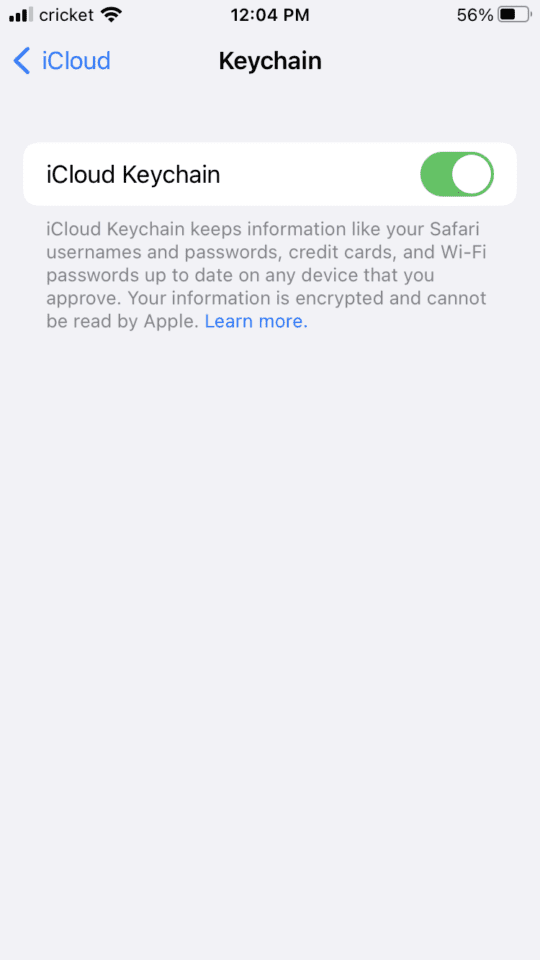The image displays a cell phone screen with a light gray background. In the upper-left corner, there are icons indicating cell reception bars, a Cricket network indicator, and a Wi-Fi signal. In the center, the time reads 12:04 p.m., and on the upper-right corner, the battery level is shown at 56%.

Beneath this top bar, there is a blue left arrow next to the word "iCloud." Centered below, in bold text, is the word "Keychain." Directly underneath is a white, thin rectangular box with black text that reads "iCloud Keychain." This option is toggled on, indicated by a green switch.

Further down, on the gray background with gray text, a description reads: "iCloud Keychain keeps information like your Safari usernames and passwords, credit cards, and Wi-Fi passwords up to date on any device that you approve. Your information is encrypted and cannot be read by Apple." Below this description, the phrase "Learn more" is presented as a blue hyperlink. The screen has no visible edges or additional buttons.